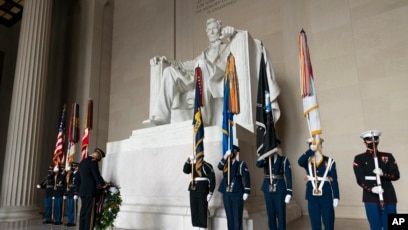The image depicts a large, white statue of Abraham Lincoln seated on a grand chair, located at the Lincoln Memorial. Flanking the statue are nine uniformed guards: five standing on the right and three on the left, with an additional guard positioned in front, bowing down towards the statue as he places a wreath. The guards are dressed in navy blue uniforms and white hats, and some wear black hats. They each carry flags, and the guards at the outer edges also hold rifles pointed straight up. The base of Lincoln's chair rises a couple of feet above the heads of the guards, highlighting the statue’s imposing stature. In the background, large columns frame the scene, adding to the monument's majestic setting. The letters "AP" are visible in the bottom right corner of the image.